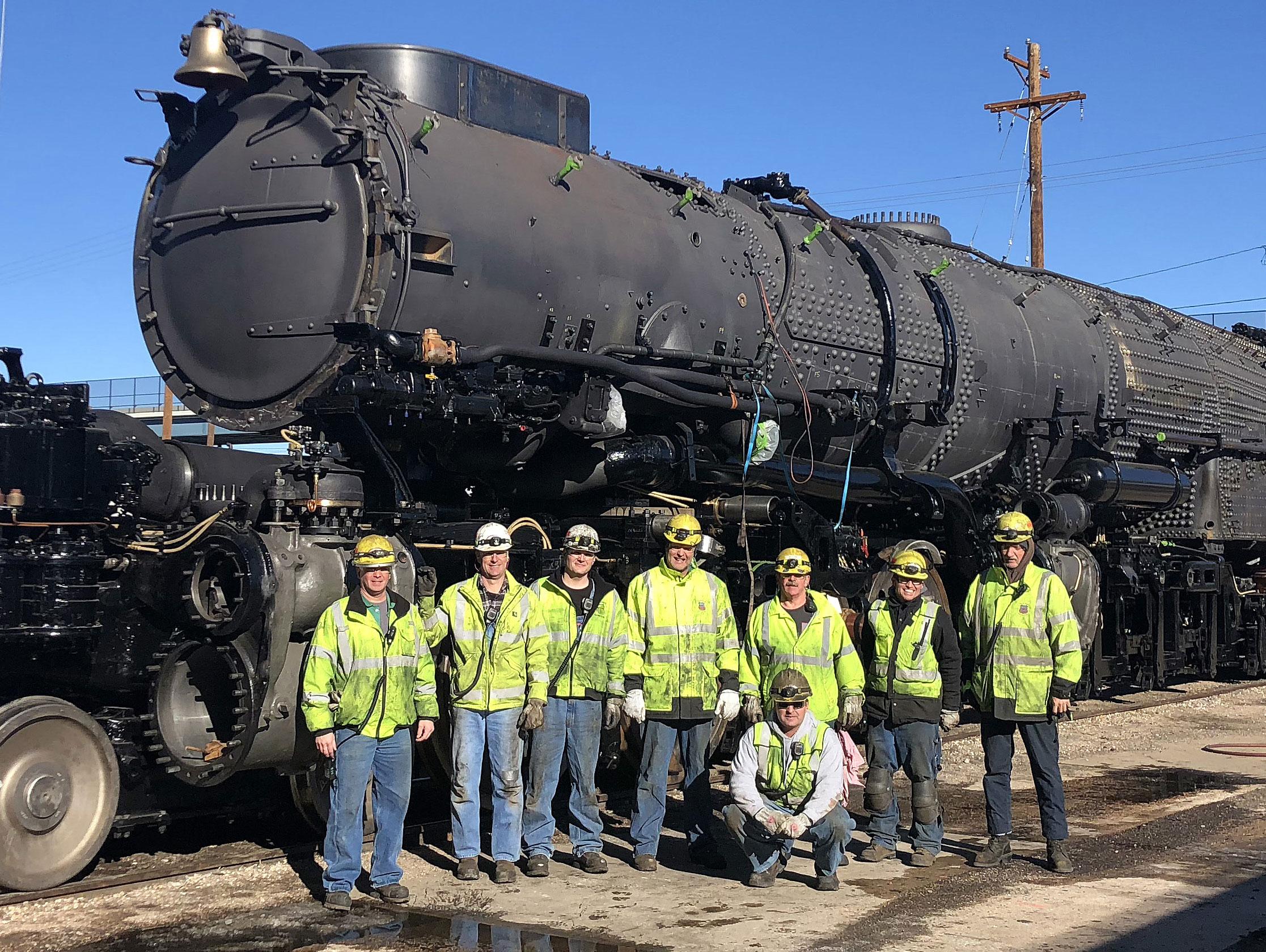In the image, eight men stand in front of a large, black, cylindrical steam locomotive on a clear, sunny day with a strikingly blue sky and birds perched on a telephone pole in the background. The men are dressed in yellow reflective safety vests with white stripes, jeans, and a mixture of yellow and white hard hats, each equipped with a lamp on the front. The locomotive, which appears partially disassembled, suggests ongoing restoration or repair, despite its old-fashioned design. The single visible train car, likely the engine, features a prominent bell at its front. The men are positioned with one kneeling at the front, possibly indicating a leader or supervisor among the group.